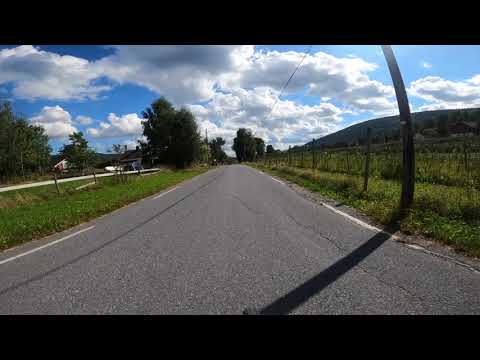The image captures a first-person perspective looking down a gray, asphalt road that stretches from the foreground to a vanishing point in the distance. Black horizontal bars frame the top and bottom of the photograph, adding a letterboxing effect. The road is flanked by grassy areas on both sides, with a slight ditch on the left. To the right, a wooden fence and a telephone pole cast a shadow across the road. In the background, a green hill rises on the right, while trees border the left, interspersed with a few small buildings and a white vehicle among them. Above, a bright blue sky dotted with puffy cumulus clouds completes the scene, giving it a serene, open-air atmosphere.